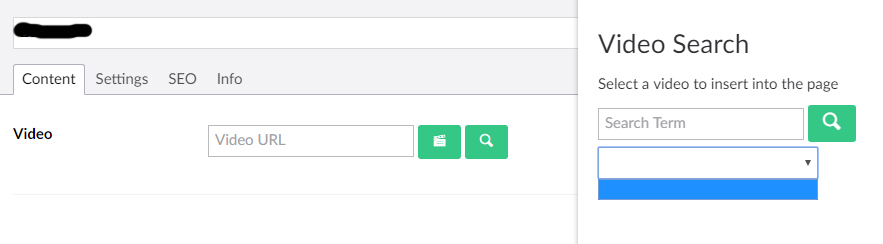The interface features a gray bar situated at the top left corner, within which a white rectangle is positioned. This white rectangle has text that has been obscured by a black marker. Adjacent to the gray bar is a white tab labeled "Content," followed by tabs labeled "Settings," "SEO," and "Info."

Below these tabs, the display includes a gray-outlined rectangle with the placeholder text "Video URL" inside it. Near this element, two green rectangles are present: one contains an indistinguishable white symbol, and the other houses a magnifying glass icon. 

A vertical gray line divides the interface. On the right side of this line, the words "Video Search" are prominently displayed, with text beneath instructing users to "Select a video to insert into the page." Further down, another gray-outlined rectangle labeled "Search Term" appears, followed by a green rectangle with a magnifying glass icon. Below these elements, a blue-outlined rectangle with a downward-pointing arrow is shown, and directly beneath this is a solid blue rectangle.